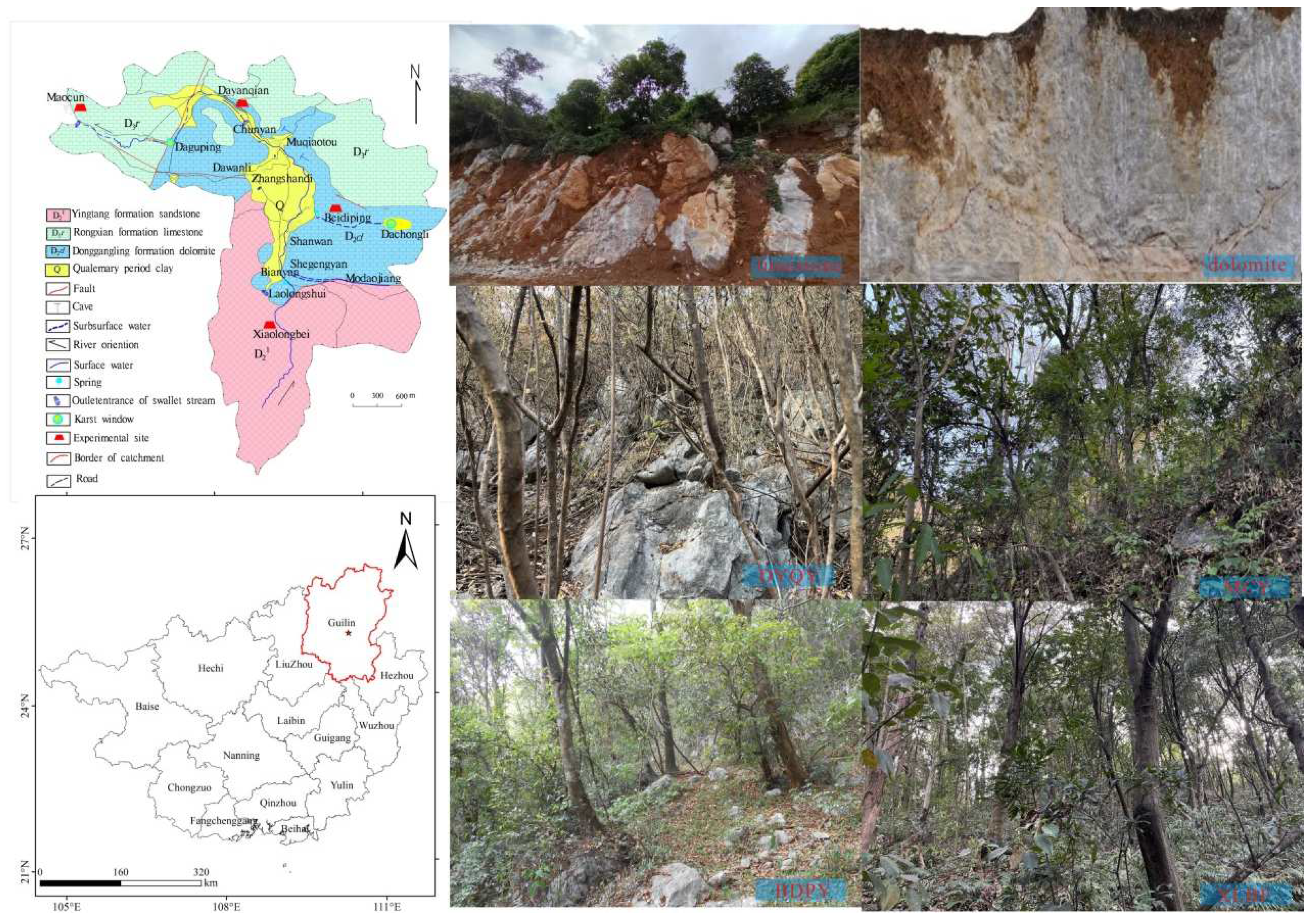The image is a composite of geographical and forest landscapes with six photographs aligned in a grid on the right side. The top two pictures depict mountain ranges with prominent gray rock formations and brown dirt, set against a backdrop of trees and sky. Below, on the left side, is an image of a wooded area with scattered gray boulders and trees without leaves, and to the right, another wooded region with sparse trees and rocks on the forest floor. At the bottom, two more photos show forest environments with small gray boulders and trees dispersed throughout.

On the left side of the image, there is a detailed, color-coded map, featuring red, green, blue, and yellow regions, indicating different rock types or geological formations. Below this map is a black-and-white diagram likely depicting a particular province in China, with a red outline highlighting a specific area. Each photograph on the right has a semi-transparent blue box with red lettering, identifying the primary rock type present in each scene. Together, these elements present a detailed overview of varied geographical features and forested environments, focusing on rock formations and landscapes.